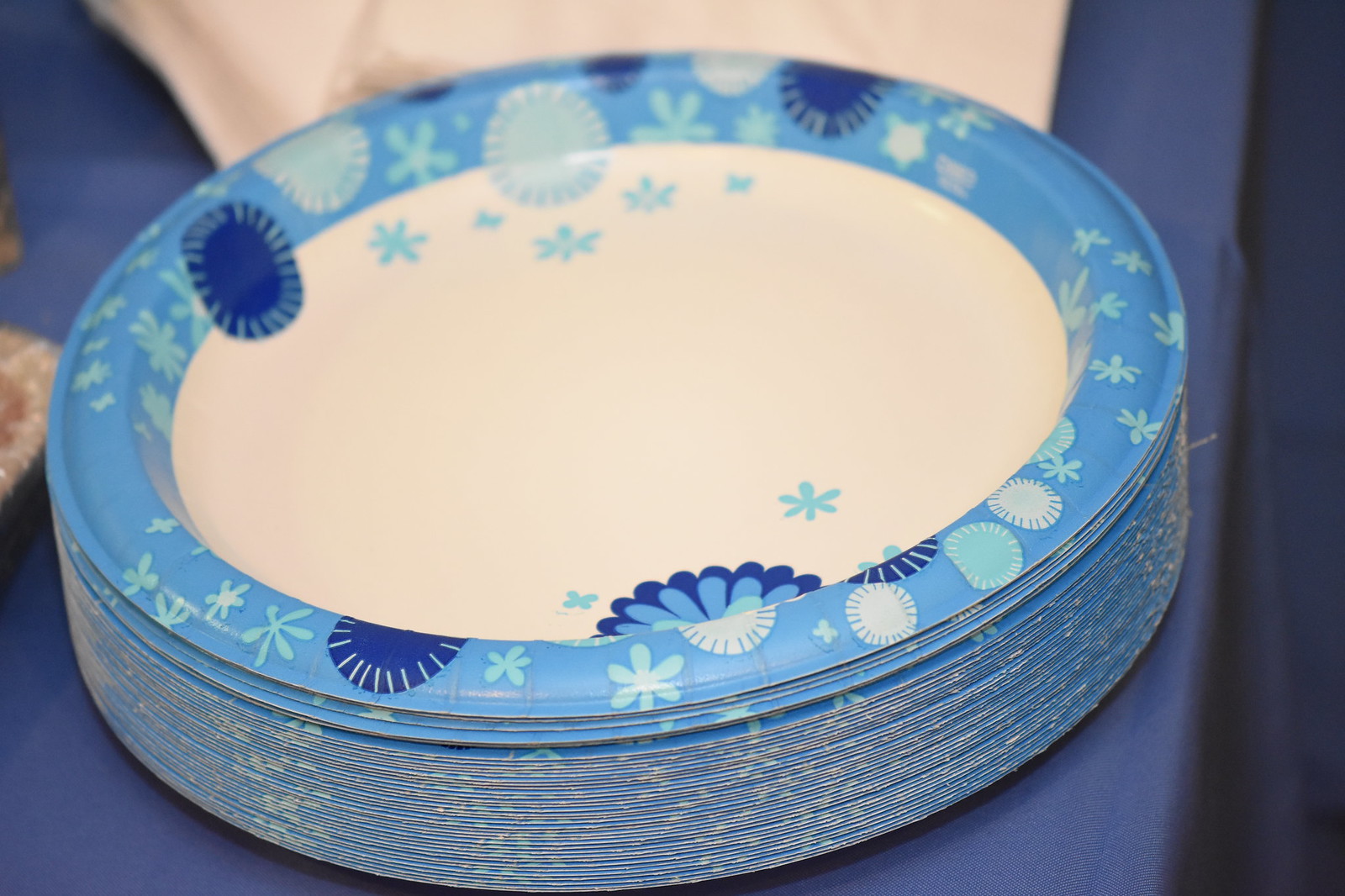This is a horizontal rectangular color photograph featuring a sizable stack of paper plates, possibly between 25 to 50, neatly piled atop one another. The plates, which have a white center, are adorned with light blue edges detailing dark blue circular and floral patterns, reminiscent of small sunflower petals and starbursts. The stack is positioned on a medium blue tablecloth, touching the bottom edge of the frame. The plates occupying the upper section of the stack appear slightly blurred due to the depth of field. In the background, there is an indistinct cream-colored item atop the tablecloth, and off to the left, a blurred object that might be an aluminum tray corner can be seen, along with something wrapped in white plastic or paper. The photo contains no writing, people, or animals, focusing solely on the detailed arrangement and design of the paper plates.